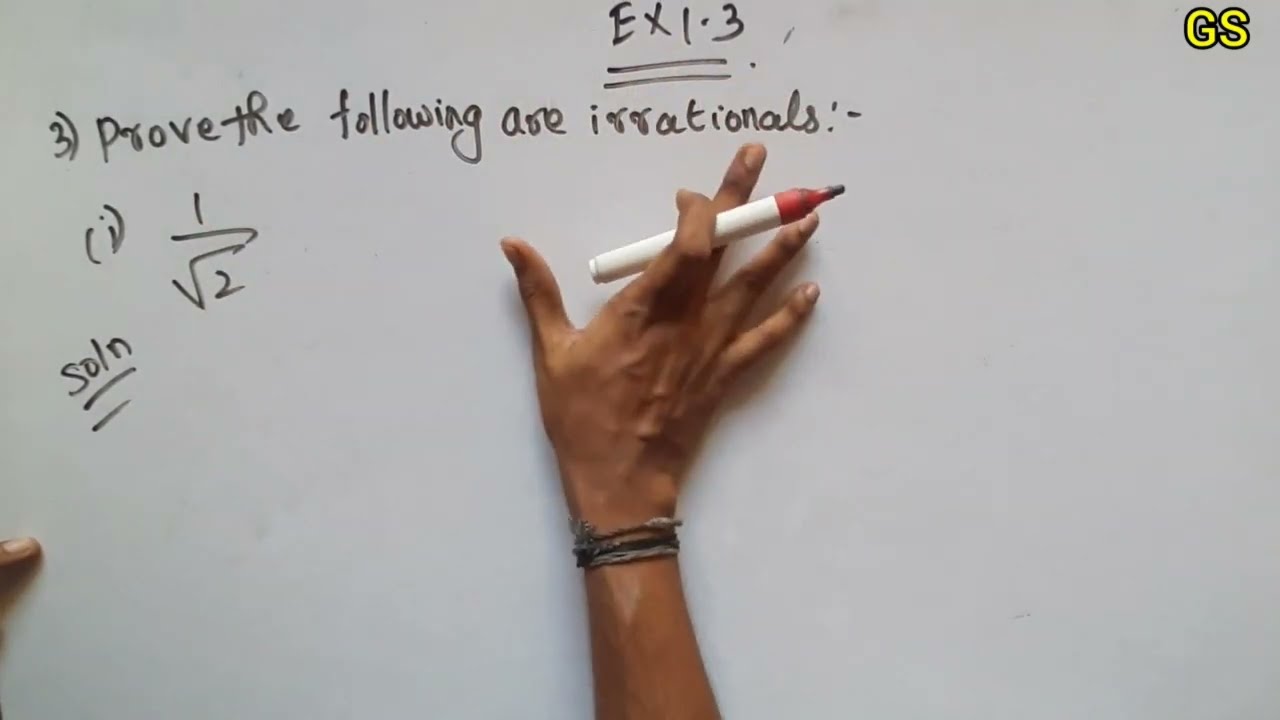A detailed photograph showcases a woman's hand reaching up and spreading out across a whiteboard. Her pointer and middle fingers clutch a red marker with a white body and red tip, poised as if underlining or about to write. On her wrist are small, woven bracelets, adding a touch of personal style. The whiteboard features multiple notations: at the top, "EX1-3" is written, indicating examples 1 through 3, with "3)" just below and to the left, followed by a mathematical instruction, "prove the following are irrationals: -". Beneath this, various equations are partially visible, including "1/2 squared." In the bottom left corner, the text "SOLN" is clearly marked with two lines under it. The top right corner of the image incorporates a computer-generated addition, displaying the letters "GS" in yellow font with a black outline. The composition is intimate, measuring approximately 8 inches wide by 5 inches tall, making the details in the photograph quite pronounced.